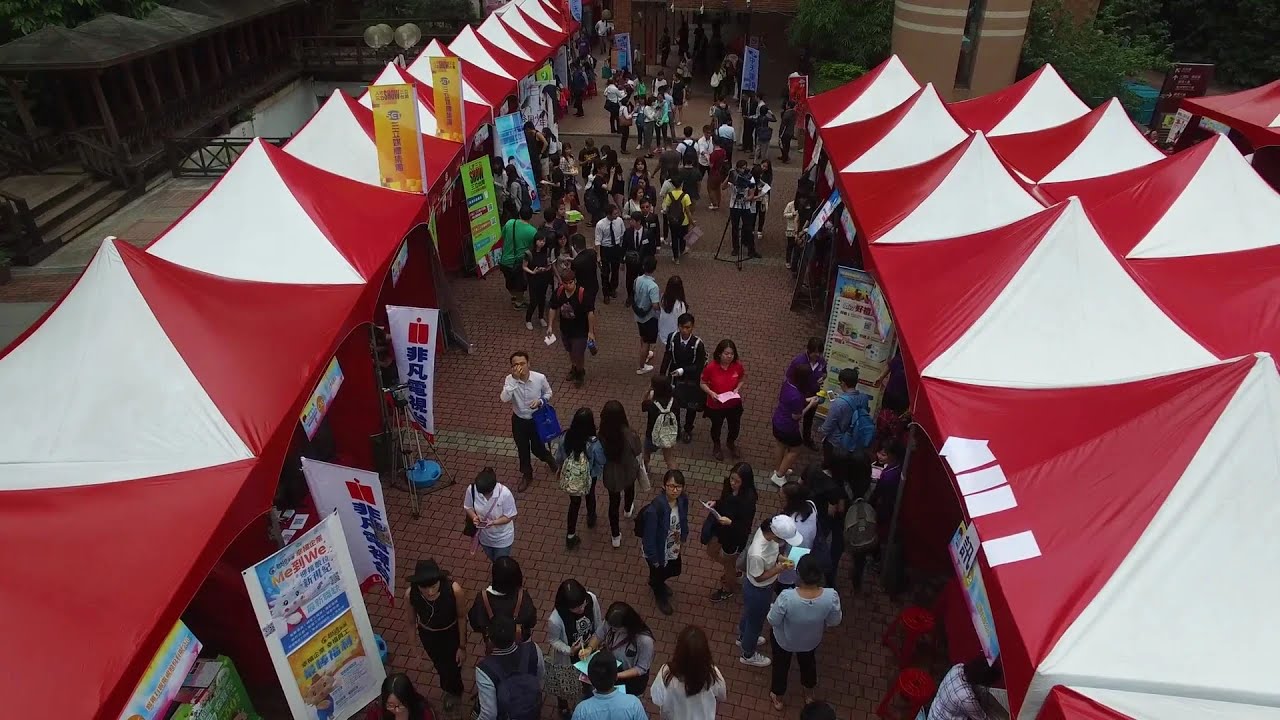This highly detailed aerial photograph captures a bustling outdoor market, staged along a central cobbled stone lane composed of red and brown stones, indicating a vivid and vibrant atmosphere. The central lane traverses the middle of the image, flanked by rows of tents on both sides. Each tent features a striking red and white fabric top, peaked in a triangular fashion, creating a uniform and festive appearance.

On the right-hand side of the central lane, an additional row of similarly topped tents stretches further towards the edge of the image, suggesting an expansive layout. Meanwhile, the left-hand side showcases several colorful banners and flags adorned with writing in either Chinese or Korean, contributing to the cultural richness of the scene. These banners vary in colors, including blue, red, white, and yellow, enhancing the visual diversity of the market.

Interspersed among the lively crowd walking down the central lane, the attendees are dressed in a mix of bright and dark-colored clothing, with an abundance of white shirts and black pants. Several individuals can be spotted carrying backpacks, predominantly in white and black. The market appears densely populated, reflecting a high level of activity and engagement.

In the top left corner of the image, there are additional structures that appear wooden with a tan or beige hue, possibly traditional seating areas or stalls, contributing to the authenticity and traditional ambiance of the scene. The background features traditional, dark brown architectural elements, further anchoring the market in its cultural setting.

The overall scene exudes the energy and cultural diversity of an outdoor fair or market, likely situated in an Asian country, as indicated by the text on the banners and signs. The overcast day bathes the market in natural, diffuse light, enhancing the clarity and details of this vibrant and crowded marketplace.